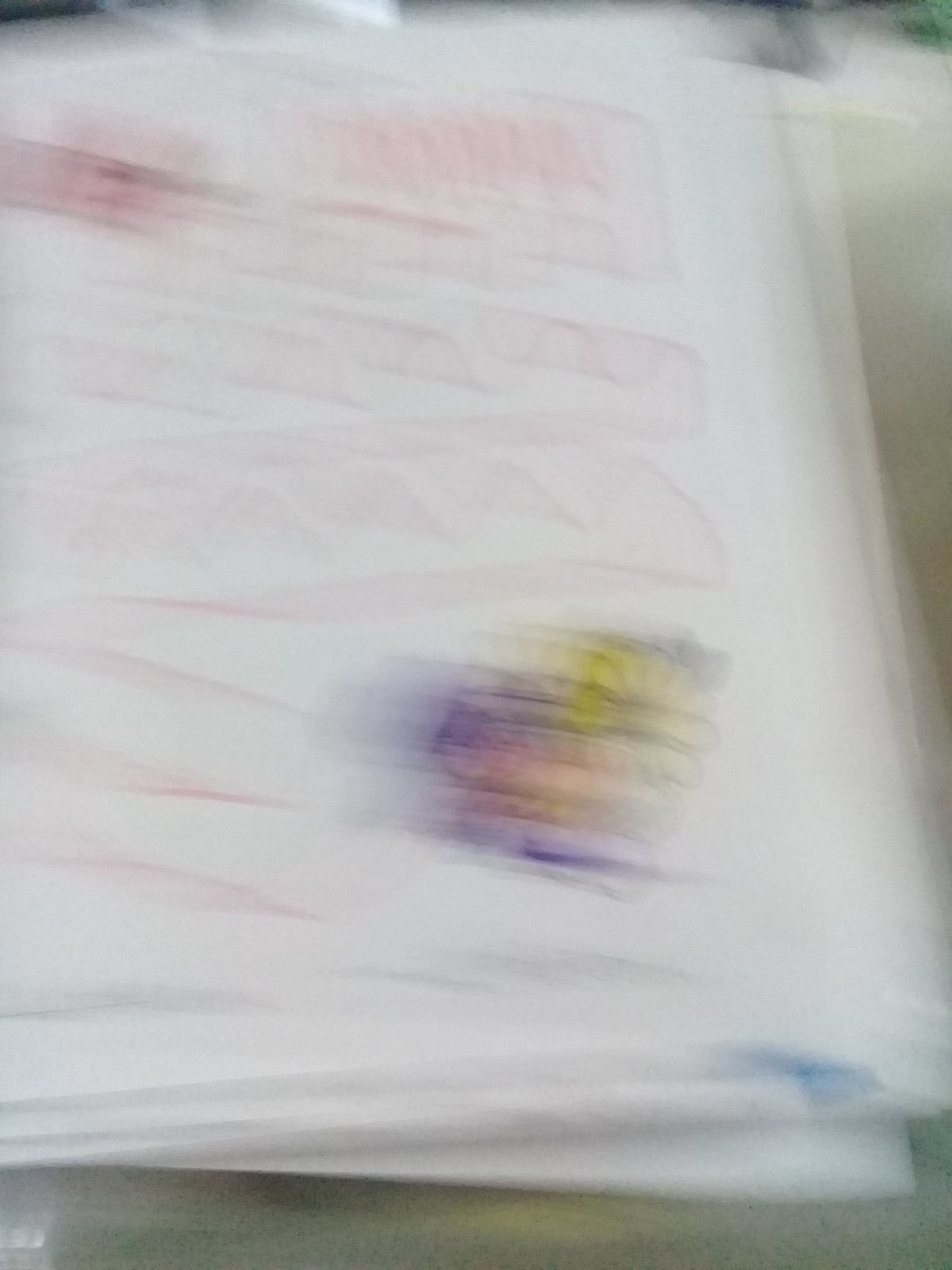This image features a completely blurry depiction of what appears to be a drawing on layered paper. The background in the upper right corner and along the bottom is primarily a grayish shade, contrasting with the predominantly white foreground. The visible layer, which seems to be the top paper layer, is covered with a pinkish-red scribble that spans across its entire surface. In the lower right corner, there is an area with a more concentrated set of scribbles in purple, yellow, and orange hues. Another denser cluster of pinkish-red scribbles is present in the upper left corner. Despite the overall blurriness, the mix of colors and scattered scribbles create a sense of chaotic vibrancy.